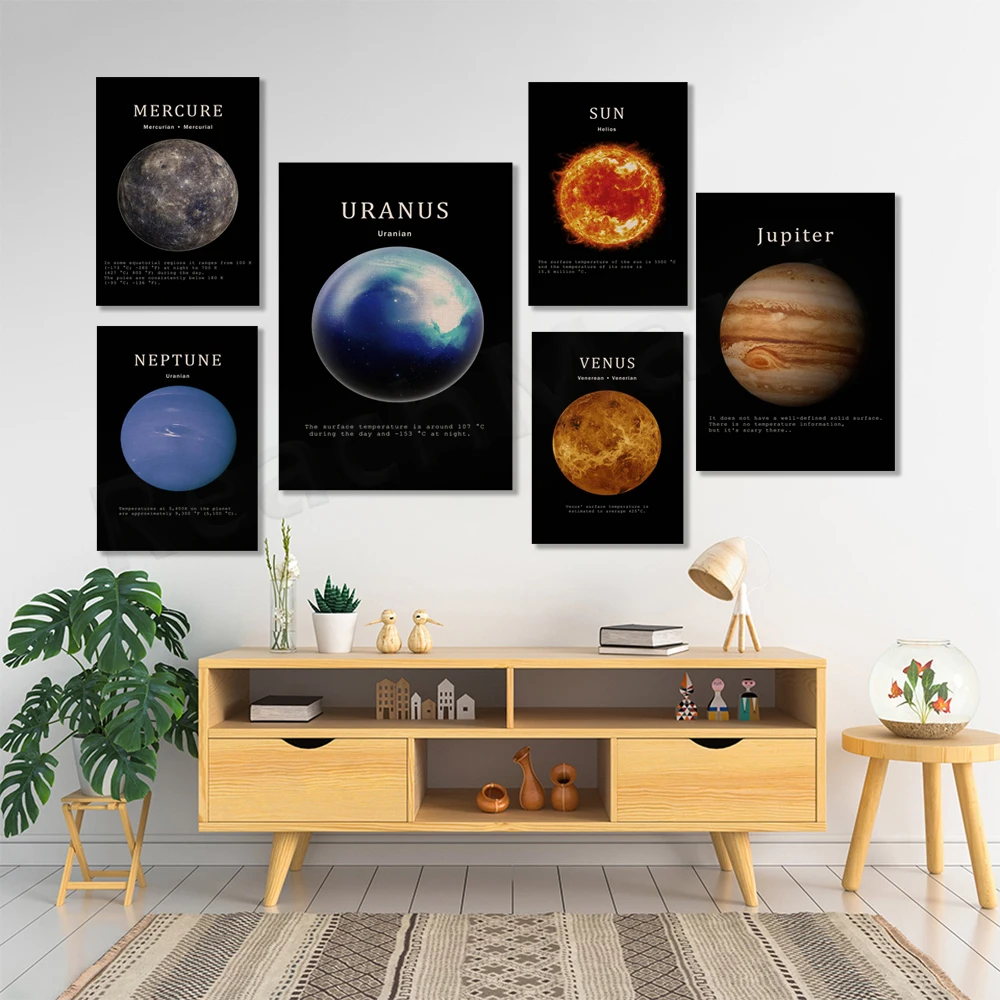This photograph showcases a meticulously designed modern living room, dominated by a prominent white wall adorned with six eye-catching posters, each featuring a different planet or celestial body against a stark black background. Arranged in a masonry-style layout, the posters depict Mercury at the top left, Neptune below it, Uranus in a larger frame to the right, the Sun and Venus stacked vertically further right, and the largest of them all, Jupiter, on the far right. The detailing of each planet is vivid, with colors ranging from blue to yellow to red.

Below these posters, a sleek light brown wooden low cabinet serves as an entertainment center. It is topped with various decorative items, including books, a lamp, and a small potted plant, adding a touch of greenery. To the left of the cabinet, a larger plant sits in a white planter, while to the right, a small stool holds a fishbowl with three fish.

The room's white wooden floor contrasts with a centrally placed beige and black rug, unifying the setting. The harmonious use of light-colored wood for the cabinet, the plant stand, and the stool enhances the room's cohesive aesthetic, making it a stylish and serene living space.